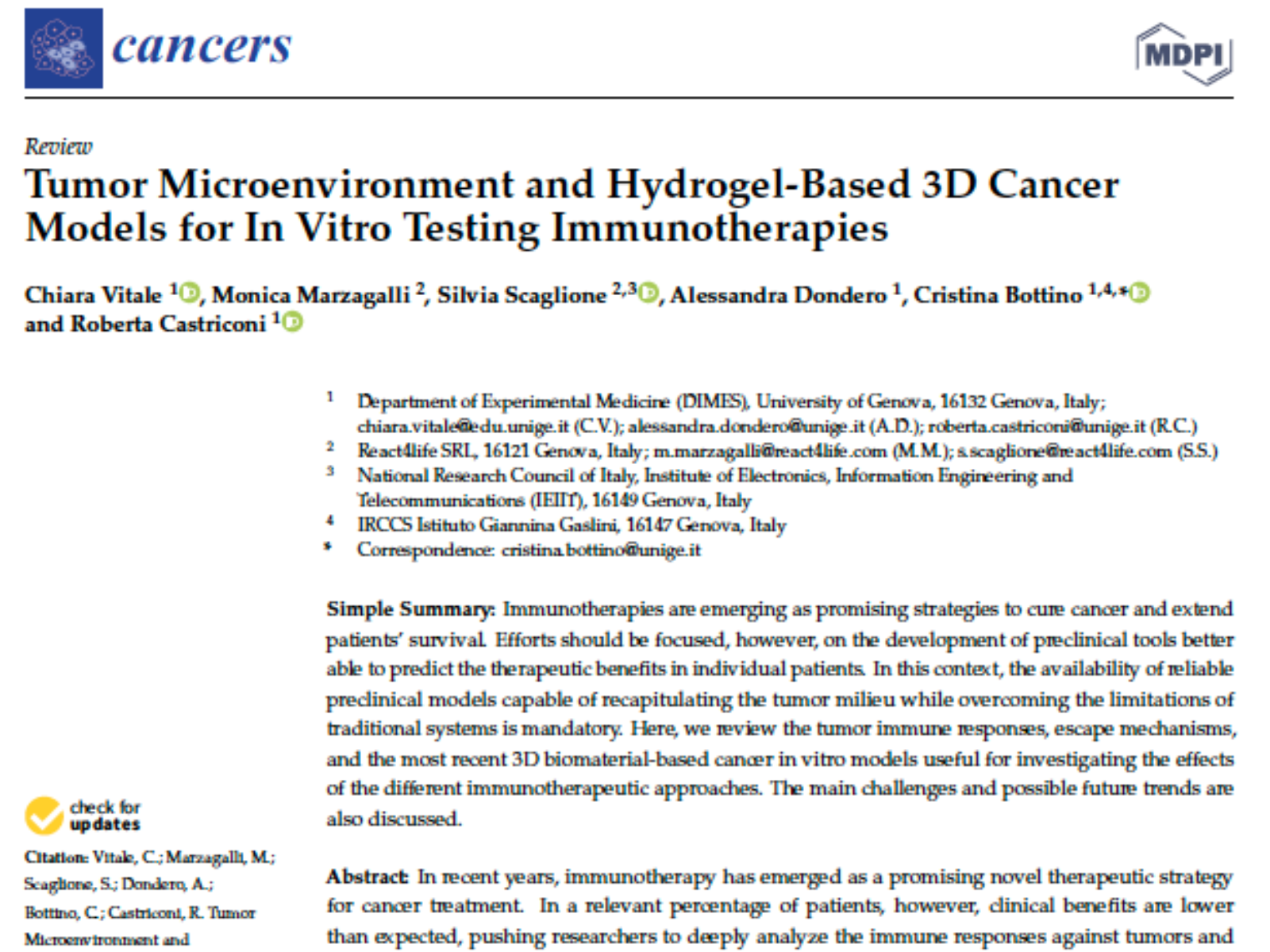This screenshot depicts a medical abstract on a white background. In the upper left corner, there is a square blue box containing cell-like drawings. To the right of this box, the text "Cancers," written in blue, is clearly visible. On the far right side, the initials "MDPI" appear, encased by angular gray lines on both sides. A long black line runs horizontally beneath this text.

Following this, the title of the abstract reads: "Review Tumor Microenvironment and Hydrogel-Based 3D Cancer Models for In Vitro Testing Immunotherapies." The authors listed are Chiara Vitale, Monica Marzagalli, Sylvia Scaglione, Alessandra Dondero, Christina Bottino, and Roberta Castricani. 

The abstract summarizes emerging immunotherapies as promising strategies to cure cancer and extend patient survival. It emphasizes the importance of developing preclinical tools that can predict therapeutic benefits for individual patients. Reliable preclinical models that can accurately recapitulate the tumor microenvironment while overcoming traditional system limitations are crucial. This review discusses tumor immune responses, escape mechanisms, and recent 3D biomaterial-based cancer in vitro models that are useful for studying the effects of various immunotherapeutic approaches. Additionally, the main challenges and potential future trends in this field are explored.